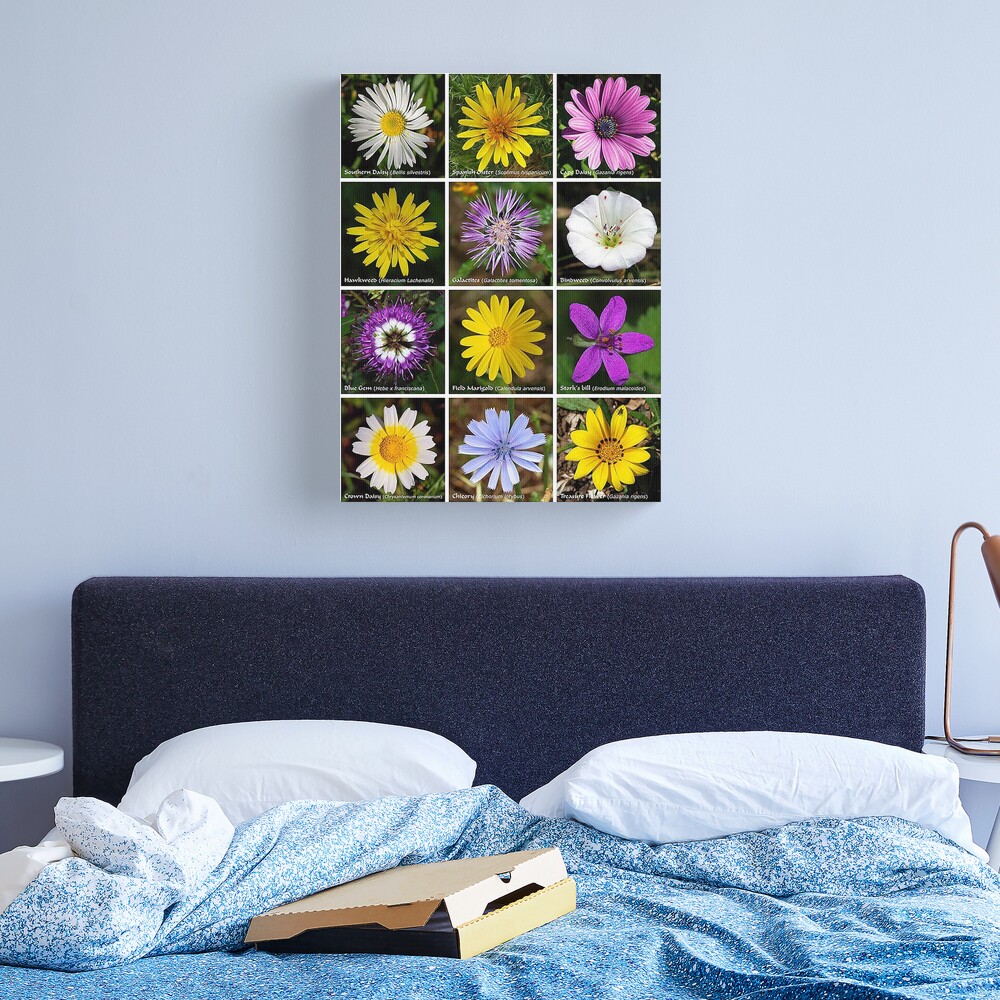In the image of the bedroom, we primarily see an unmade bed adorned with baby blue sheets featuring white designs. Atop the bed, there is an open box, likely a pizza box, suggesting casual usage. Above the bed, the wall—painted in a light pastel blue—displays a framed picture featuring four rows of flowers. These flowers include various pastel hues: purple, white, pink, and even some daisies among them. Additionally, there is a small lamp positioned on a bedside table, adding a cozy element to the scene. Overall, the room exudes a casual, lived-in vibe without appearing messy or unclean.